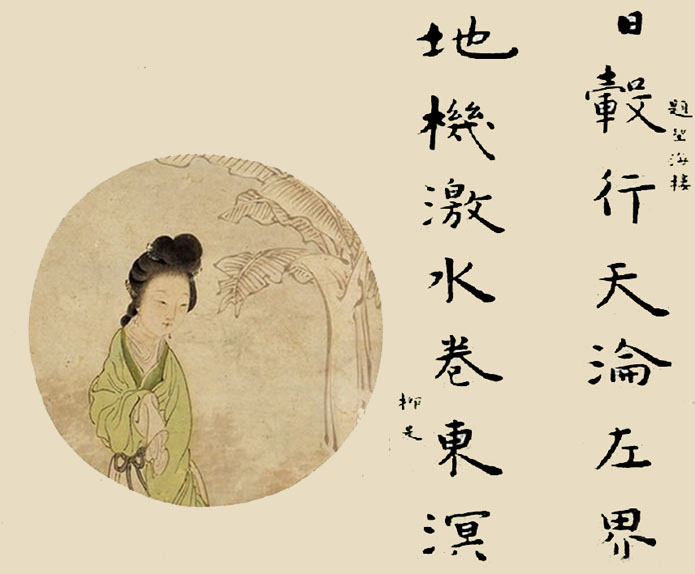The image is a detailed Chinese painting set against a beige background. On the left side, a prominent light brown circle features an ancient Chinese woman dressed in a traditional long green robe with very long sleeves, her black hair styled in several ornate buns. Adjacent to her, within the circle, stands a small tree or plant. The right side of the painting displays three rows of Chinese characters in black ink. The left row reads "地击击水卷东铭," the middle row states "日谷行天论左界," and the rightmost row says "提灯海流." This intricate artwork blends traditional iconography with precise calligraphy, offering a glimpse into ancient Chinese culture.